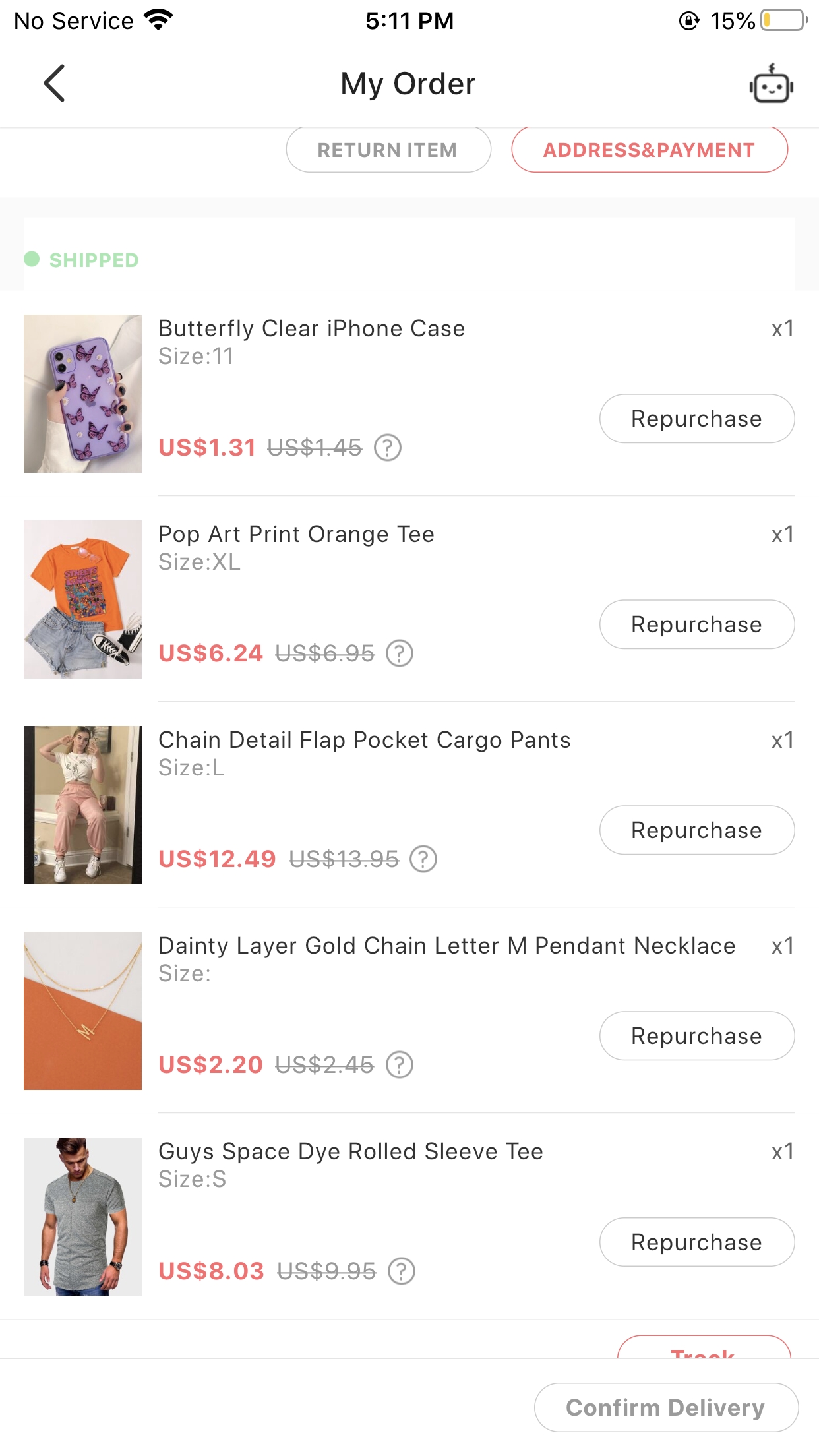**Website Category: Order Summary**

The screenshot displays an order summary page on a phone with 'No Service' indicated at the top left, timestamped at 5:11 PM, and showing the battery level at 15%. A back arrow is visible for navigation. The top bar reads "My Order" and features a small robot face icon.

Below the header, options for "Return Item" and "Address and Payment" are available, followed by a section labeled "Shipped".

1. **Butterfly Clear iPhone Case**:
   - Size: 11
   - Price: US $1.31
   - Quantity: 1
   - Option to repurchase available.

2. **Pop Art Print Orange Tee**:
   - Size: XL
   - Price: US $6.24
   - Quantity: 1
   - Image shows the tee alongside a pair of shorts and black sneakers.
   - Option to repurchase available.

3. **Chain Detail Flap Pocket Cargo Pants**:
   - Size: Large
   - Price: US $12.49
   - Quantity: 1
   - Image features a person wearing the cargo pants.
   - Option to repurchase available.

4. **Dainty Layer Gold Chain Letter 'M' Pendant Necklace**:
   - Price: US $2.20
   - Quantity: 1

5. **Guy's Space Dye Rolled Sleeve Tee**:
   - Price: US $8.03
   - Quantity: 1